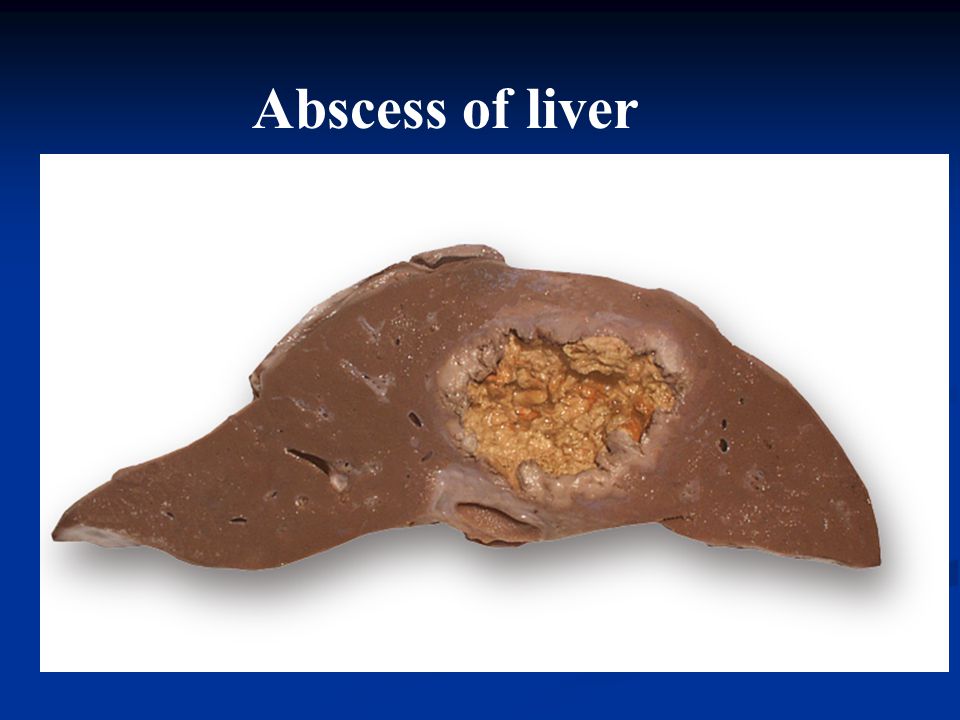This image serves as an educational infographic, presumably from a medical PowerPoint presentation. It features a detailed photograph of a liver affected by an abscess, prominently centered against a predominantly white background, with an outer blue border. Above the image, the text "Abscess of Liver" is displayed in white on a blue background. The liver, brown with various shades including lighter brown and orange, exhibits a distinct cross-section that is detailed and textured. The affected area appears granulated and contains yellowish-brown regions with noticeable holes, lending a somewhat unusual and intricate appearance to the organ. The overall setting and composition suggest a clinical or educational context, aiming to illustrate medical conditions actively, possibly as part of a classroom or technical training.